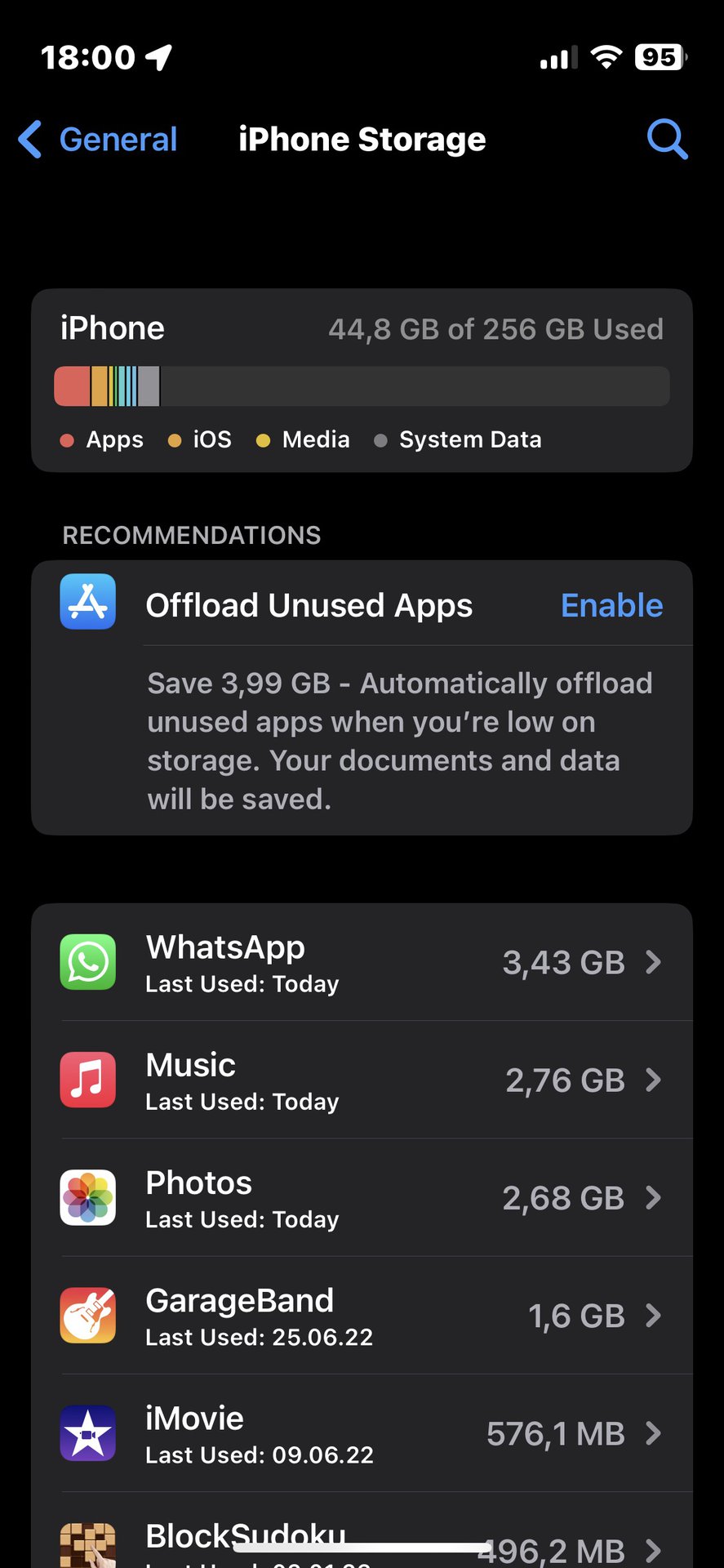The image resembles the interface of an iPhone, displayed in a vertical format akin to a phone screen. In the upper left corner, the time reads "18:00" in white text, accompanied by a white arrow pointing to the right. The upper right corner features standard iPhone status icons: the Wi-Fi signal, cellular reception bars, and a white battery icon displaying "95" in black text, indicating the battery percentage.

Below the status bar, the page has a black background. At the top center, "iPhone Storage" is written in white text. To the left, highlighted in blue, is the word "General," and to the right, there is a blue magnifying glass icon, indicating a search function.

Beneath this section, in a gray box, the text "iPhone" appears alongside a storage summary saying "44.8 GB of 256 GB used." Below this, there is a horizontal bar graph divided into different colored segments, representing categories such as Apps (red dot), iOS (orange dot), Media (yellow dot), and System Data (gray dot).

Further down, a section titled "Recommendations" suggests the option to "Offload Unused Apps," with an accompanying "Enable" button.

Following this, there is a list of apps sorted by storage usage. Each app entry includes its name, the last time it was used, its storage size, and its icon. The apps listed include WhatsApp, Music, Photos, GarageBand, iMovie, and Block Sudoku.